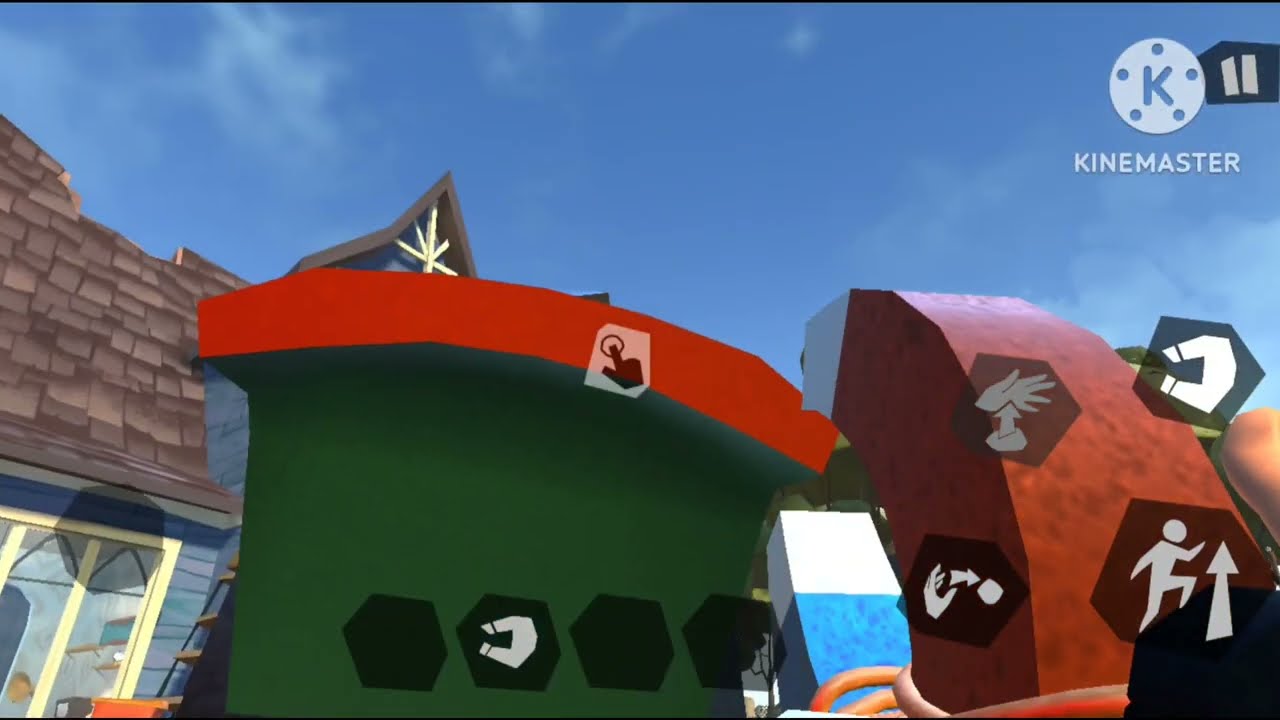This image is a screenshot from a 3D video game with a style reminiscent of the Nintendo 64 era, captured and hosted on KineMaster, as indicated by the logo and pause button in the top right corner. The scene features a large, house-sized green object with a curvy red top resembling wood, situated in the center. To the left, there is a house with blue siding, white-framed windows, and a roof made of light and dark gray shingles, giving it a cartoony appearance. The background reveals a clear blue sky.

The gameplay interface includes various control icons distributed across the screen. At the bottom, there are hexagram-shaped icons representing different game functions. Specifically, in the lower right, there are icons for a hand with an arrow beneath it, a magnet, a person with an upward arrow, and a hand in a throwing motion. In the bottom middle is a selection menu displaying a magnet as the currently chosen item. Additionally, the player appears to be interacting with the large green object using a magnet, which is red on the top, blue on the bottom, with white tips.

Overall, the detailed interface and vivid cartoony graphics suggest a dynamic and engaging gaming experience.